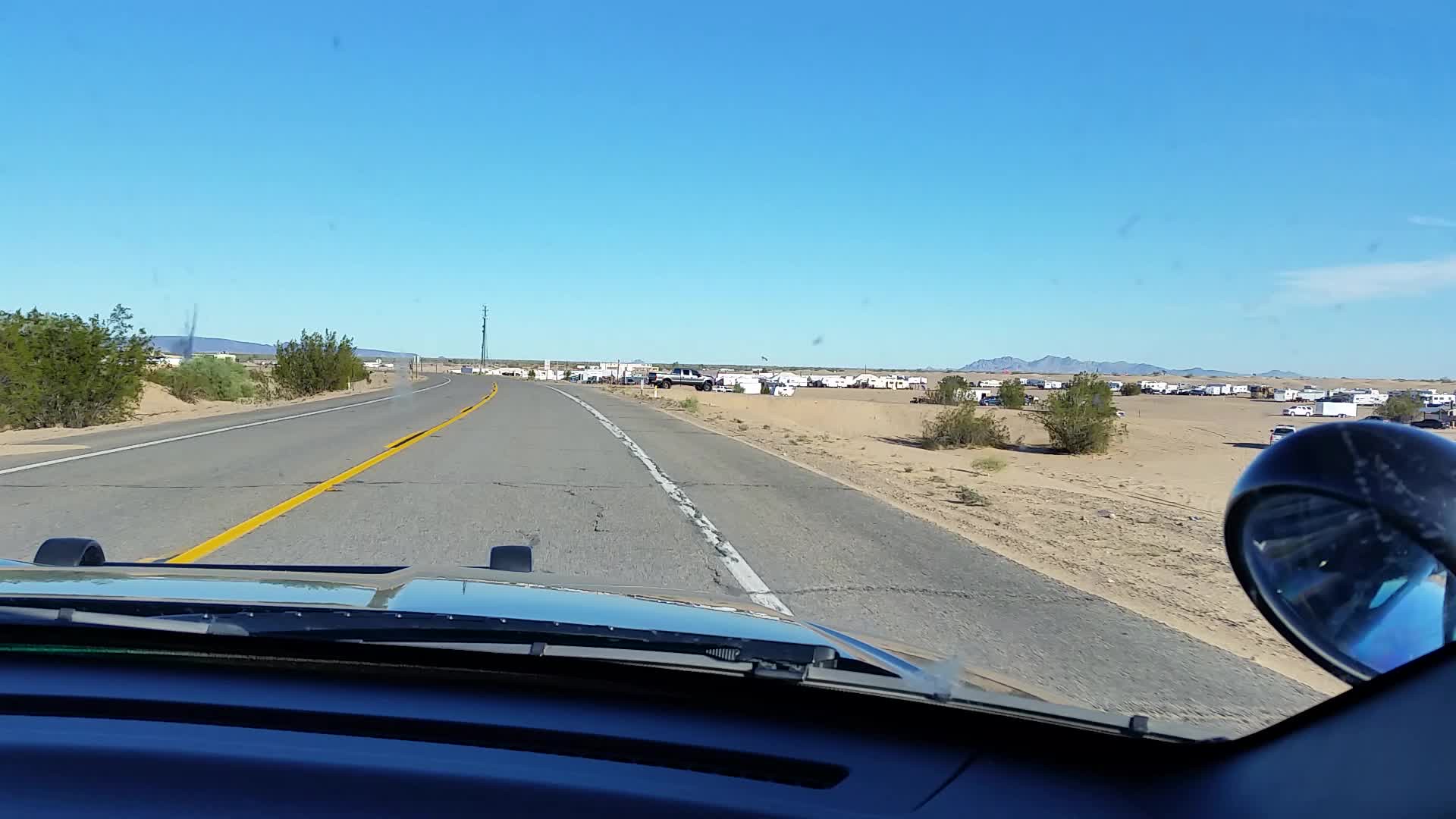The image captures the view from inside a moving vehicle, likely a dark-colored car, evidenced by the visible front hood and a circular side-view mirror in the bottom right corner. The main focus of the image is an open, black paved road bordered by white and yellow traffic lines—yellow lines in the middle and white lines on either side. This road seems to cut through a desert-like terrain, characterized by light gray dirt, green bushes, and occasional trees on both sides. On the right side of the road, there are several small white structures, possibly homes, campers, or tents. The expansive, clear blue sky stretches across the background, adding to the vast and open feel of the scene. The road, which appears to be a major interstate, possibly in the Midwest or West Coast, is accented with minor cracks and imperfections, contributing to the rugged, scenic atmosphere.